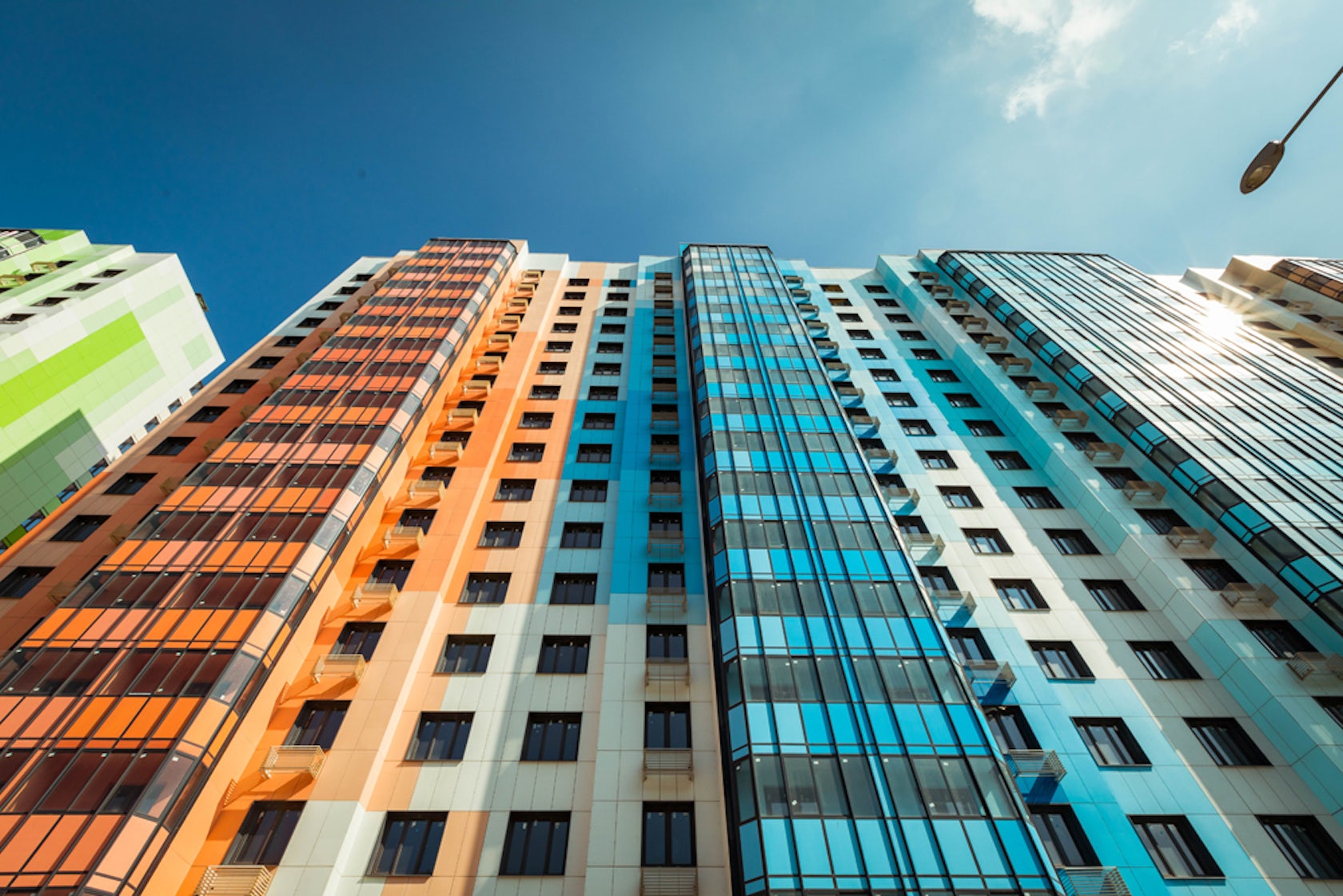This image is a vibrant, upward-looking view of a colorful, modern skyscraper composed of multiple vertical panels in various bright colors. The building prominently features green on the far left, transitioning to orange, and then multiple shades of blue towards the center and right. A clear, blue sky with a single cloud stretches above the skyscraper, adding to the vividness of the scene. A streetlight extends from the sidewalk at the bottom right of the frame, emphasizing the street-level perspective. The sun reflects off one of the blue panels on the right, highlighting the sunny weather of this city setting. The skyscraper, likely around 20 stories tall, is striking due to its multicolored facade, including bright tones of green, blue, orange, yellow, along with subtle hues like lime green, ocean blue, and creamish beige. The overall impression is one of a vibrant, contemporary cityscape.